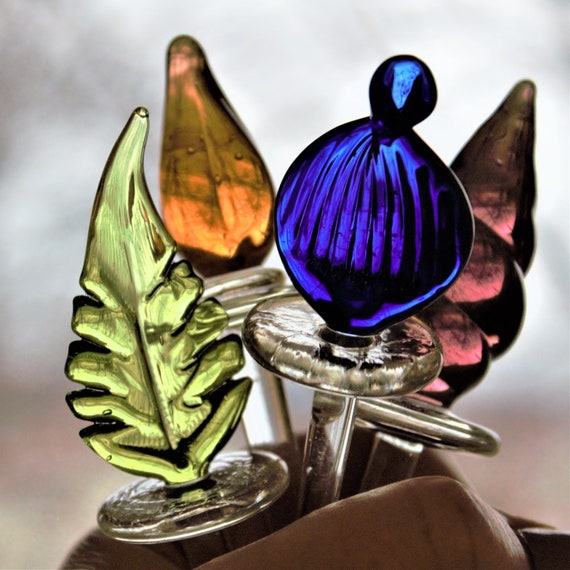The image showcases an array of uniquely shaped and colorful glass objects, each resting in individual slots carved into what appears to be a stone base. In the center and most prominent is a striking cobalt blue glass piece featuring a spherical shape with another, smaller sphere perched atop it, reminiscent of the domed towers found in Russian architecture. Moving to the bottom left, there's a delicate light green glass object shaped like a leaf, detailed with black veins running through it. In the top left portion, an eye-catching amber-colored teardrop form can be seen. Further to the right in the background, a dark purple or amethyst-colored piece catches the light, its curved, almost cone-like shape adding depth to the display. Towards the back right, there's a rose-colored object with black accents, resembling a pine cone. Each object’s handle, likely designed as a letter opener, is distinct and appears meticulously crafted. The juxtaposition of the seemingly photographic base with the potentially painted backdrop adds an intriguing layer to the overall beauty and mystery of the scene.